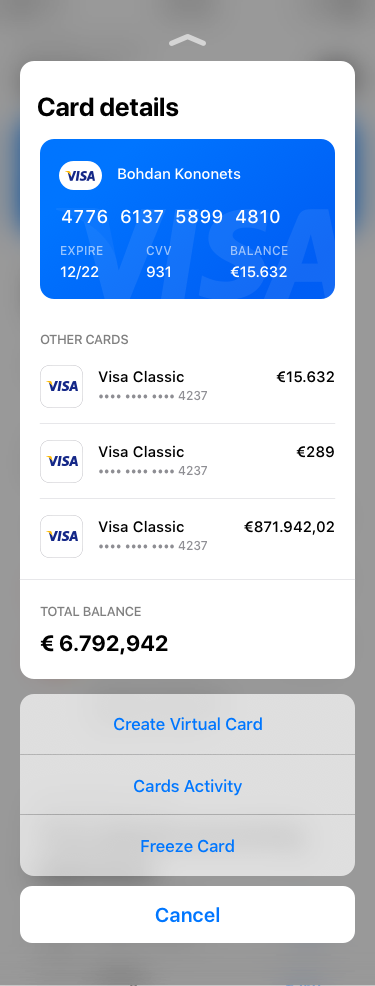This detailed graphic, sourced from a Pinterest site showcasing "39 App Bank Ideas for Mobile App Design," illustrates a mobile banking interface with a focus on card details. The primary design element features a clean white background with a grayish border encasing it, resembling the display size of a typical smartphone screen.

At the top, the section labeled "Card Details" is prominently displayed in black text. Below, a blue Visa card is portrayed, featuring the cardholder’s name, Bohdan Kononets, and the card number 4776 6137 5899 4810. The card's expiry date is 12/22, and the CVV is 931. The displayed balance for this card is £15,632.

Further down, the interface lists additional cards with summarized information:

1. Another card ending in 4237, sharing the same balance of £15,632.
2. A Visa Classic card, also ending in 4237, with a balance of £289.
3. Another Visa Classic card, again ending in 4237, showing a balance of £871,942.00.

Aggregated at the bottom of this white box is the total balance amounting to £6,792,942.

Beneath the main section, a row of gray boxes offers various functionalities, including "Create Virtual Card," "Card Activities," "Freeze Card," and a "Cancel" button, providing interactive options for the user.